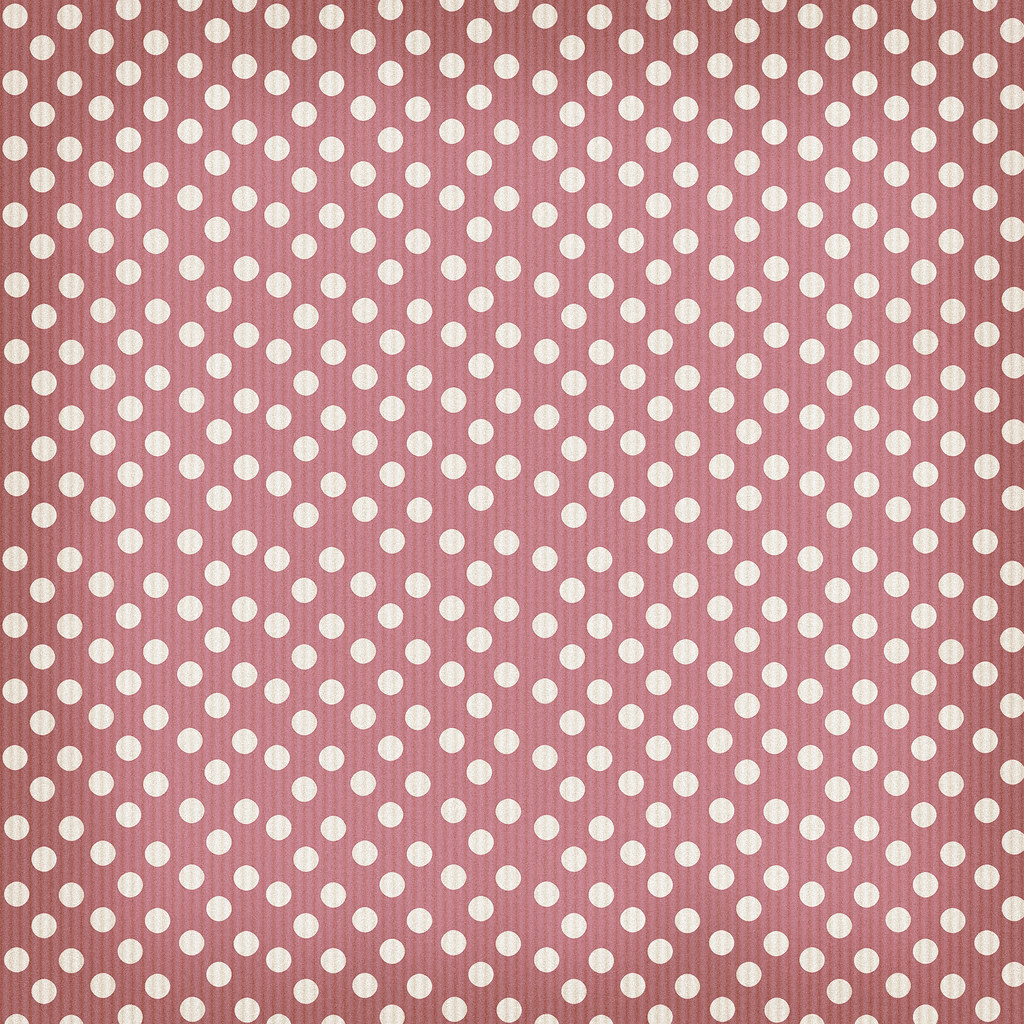The image is a detailed, rectangular graphic with a soft red background transitioning to a darker red toward the edges. It features numerous tightly-spaced, small white polka dots evenly distributed across the entire image, with likely over a hundred dots in total. Adding to the complexity, there are several very thin, closely spaced vertical lines that subtly run from top to bottom, contributing to a textured appearance. This design could resemble fabric, wallpaper, a tablecloth, or simply a digitally created graphic pattern.